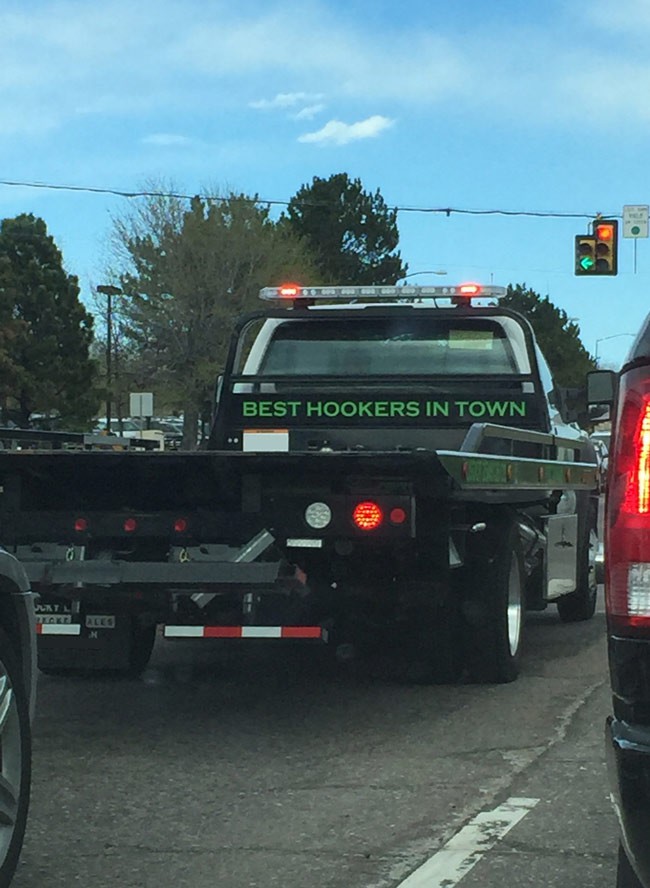In this vivid, full-color photograph captured on a mostly sunny day with a few wispy clouds in a blue sky, the central focus is a flatbed tow truck. The tow truck, featuring a white front and a black bed, faces away from the camera toward a traffic light. Prominently displayed on the back of the truck in green writing is a humorous sign that reads, "Best Hookers in Town." The truck is equipped with a light bar above the roof, where two red lights are illuminated. The tow truck's red brake lights are also on, and it has distinctive white and red stripes across the bottom behind the rear wheels. 

The truck is stopped at a traffic corner where a standard three-colored traffic light shows red on the right side, while a separate two-symbol traffic light displays a green arrow pointing left. The cracked, black-paved road is marked with a white dotted line. To the right of the tow truck, just within the frame, the back taillight of a black SUV glowing red is visible. In the background, tall trees stand under the clear sky, contributing to the scene's calm, picturesque quality.